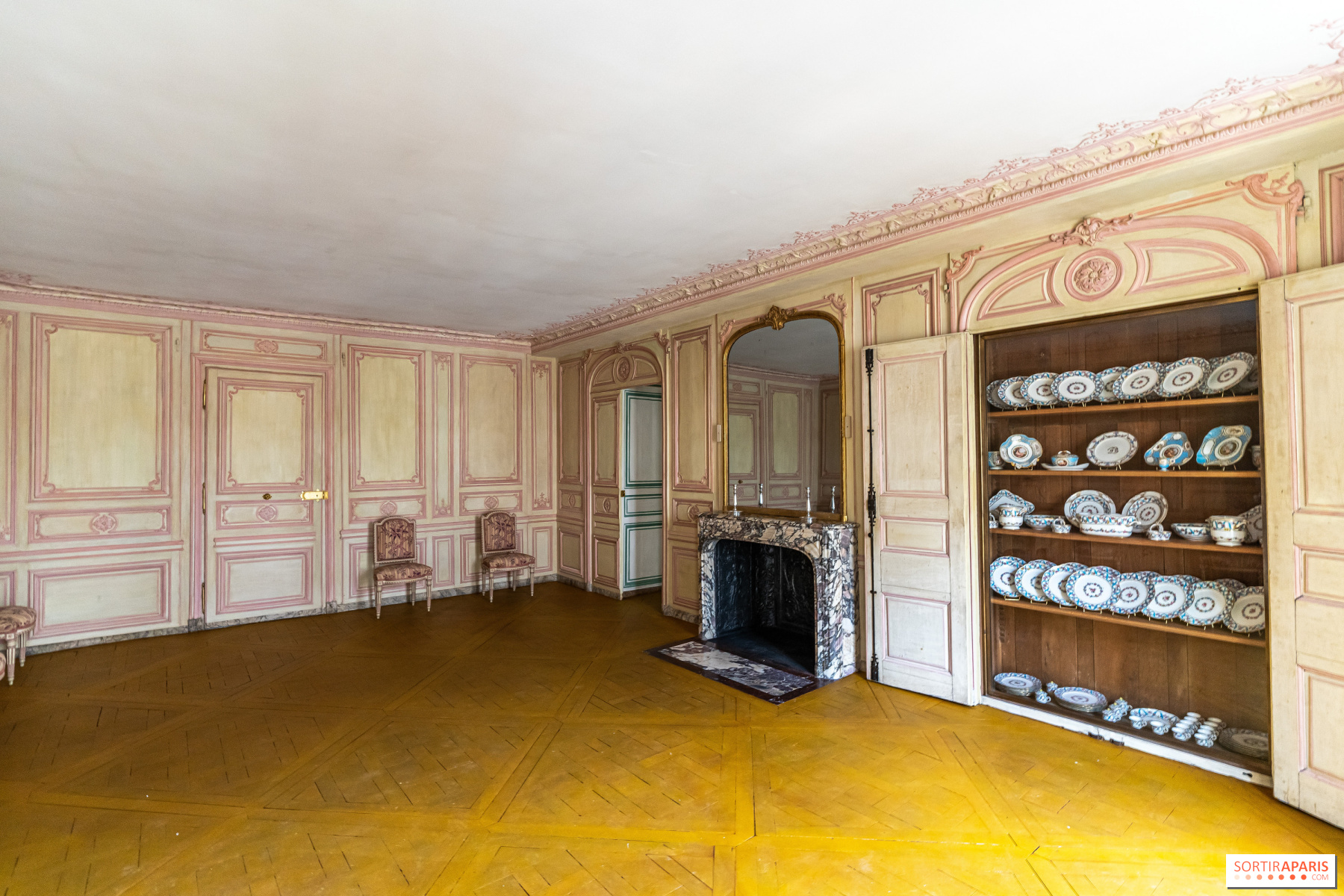The image depicts an interior space, likely a living room or a room in an old manor or hotel. The floor is yellowish wood, and the walls are predominantly white with pink trim, giving the room a distinctive two-tone appearance. The white ceiling contrasts subtly with this color scheme. Central to the room is a marble fireplace without any fire or firewood, which has a mirror above it, contributing to a slightly ominous atmosphere. To the immediate left of the fireplace is a doorway, and further along the same wall, another doorway can be seen.

On the right side of the image is a closet, or china cabinet, its doors open to reveal numerous plates and bowls, some of which are blue and white fine china. Two pink chairs are positioned against the wall to the left side of the room, indicating very sparse furniture. The overall scene suggests an abandoned or seldom-used space, reinforced by the minimal furniture and the peculiar caption "Sortir Apares" in a white box with orange lettering seen at the bottom right of the image.